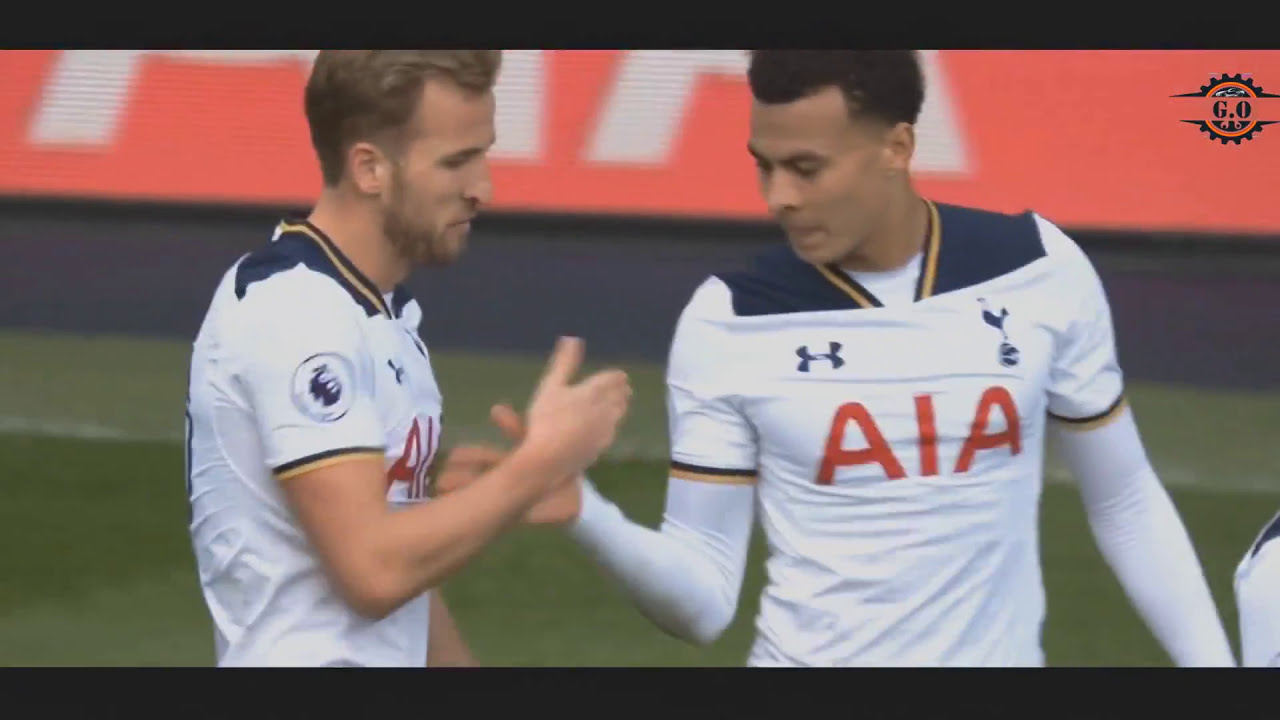A slightly pixelated image, possibly a screen grab from a TV or laptop, shows two soccer players in the middle of a high-five on a grassy field, bordered by a track. Both players wear white jerseys with blue shoulders and the word "AIA" in bright red lettering across their chests. The African-American player on the right is lean with short hair and is turning to face his Caucasian teammate, who has brown hair and a short beard. The players appear to be in motion, their hands just about to touch. Visible logos on the jerseys include navy Under Armour and Hanes. Behind them, a blurred background features billboards and a video screen with "AIA" in white lettering, framed by a salmon-colored top and a dark blue bottom.